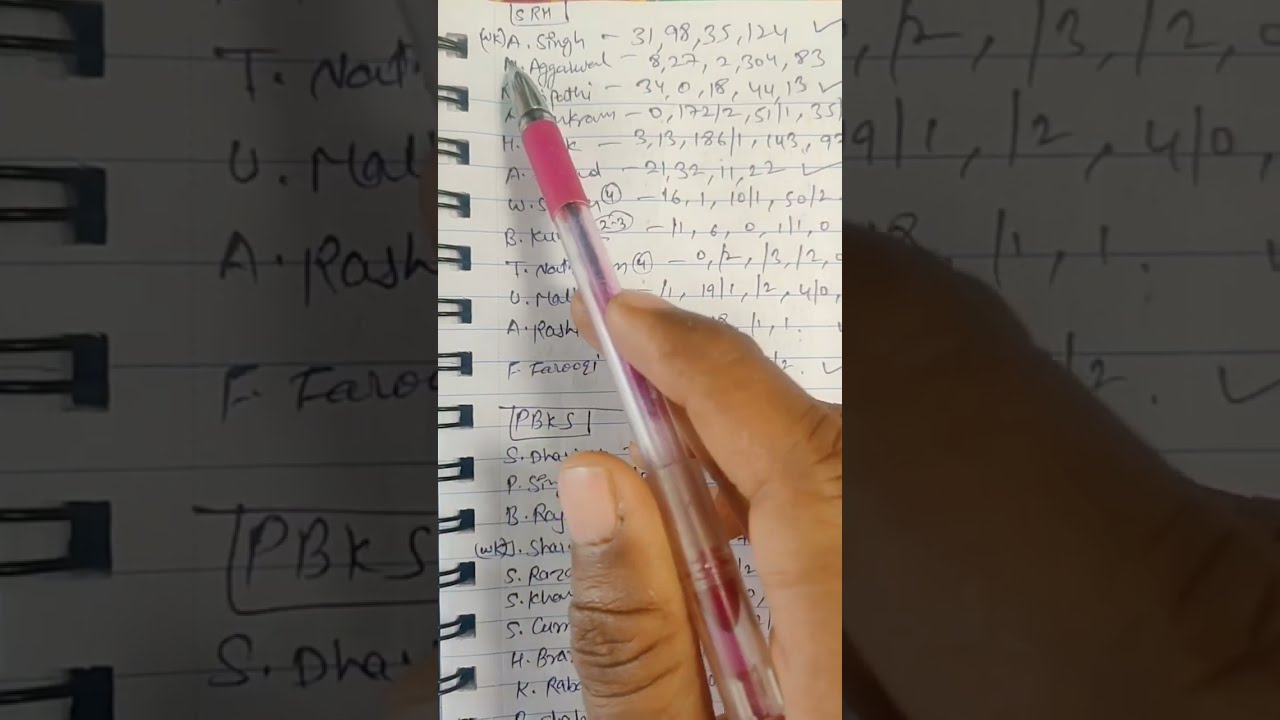The image is a detailed close-up shot of a sheet from a spiral ring notebook, extensively filled with writing. Dominating the center of the composition is a pink and silver pen, gripped in a caramel-colored right hand, poised over the paper. The pen's blue ink has inscribed several lines of text, which include a list of people's initials followed by last names and sequences of numbers. Notably, the first visible line reads "A Singh - 31,98,35,124," and another nearby line lists "M Agarwal - 8,27,2,304,83." The entire sheet appears to be densely packed with these entries, suggesting a meticulous record of scores or data of some kind. The white of the paper contrasts starkly with the darker ink, adding a crispness to the handwritten details. This scene captures the essence of someone engrossed in documenting important information in their notebook.